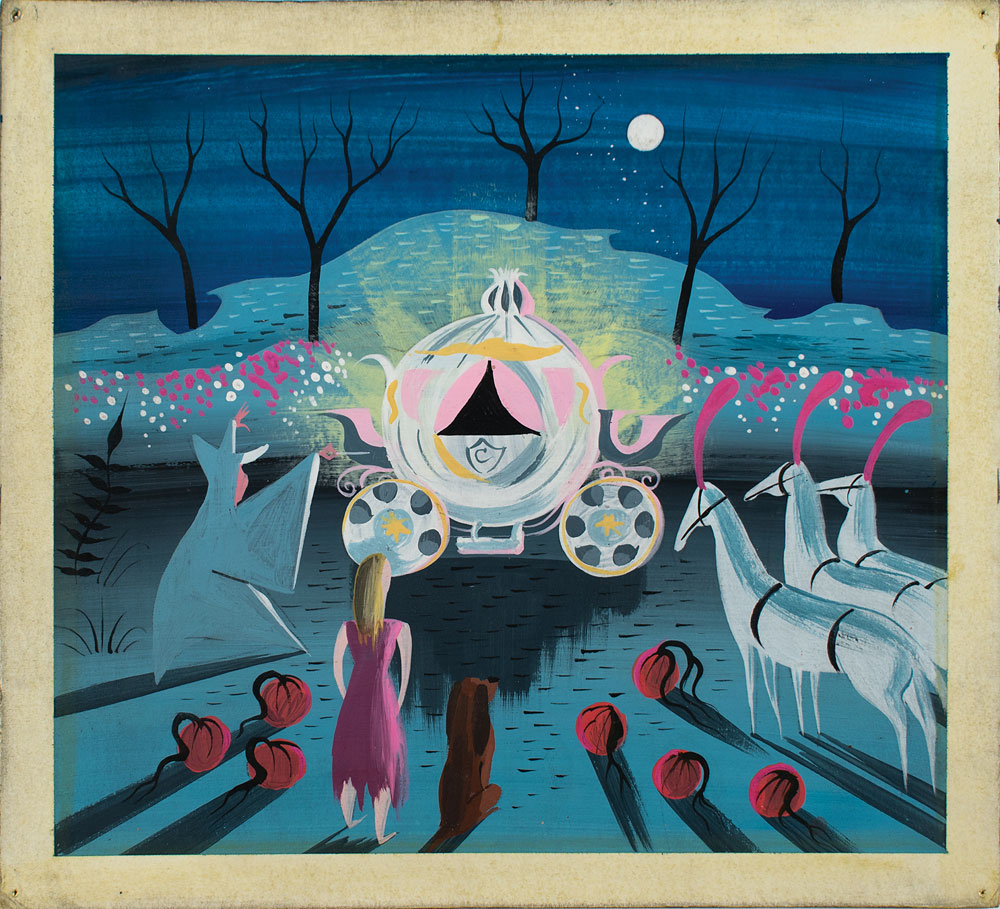This vibrant, square, cartoon drawing of a classic Cinderella scene is bordered by a light brown frame and set outdoors under a starry night sky with a full moon. The background portrays a rich tapestry of flowing hills, dense trees, and delicate flowers. The centerpiece is a magical, pink and black round carriage with four wheels, sparkling as it's being enchanted by the fairy godmother positioned to the left. This good witch, draped in a long gray robe, waves her magic wand to transform pumpkins into chariots. Cinderella, dressed in tattered pink rags, stands in front of the carriage, flanked by three pumpkins on her left and four on her right. Additionally, there's a brown dog sitting loyally next to her. On the lower right, three elegant, white horses with pink feathers in their bridles await to draw the carriage, intently gazing at it in anticipation. The detailed scene captures the magical moment of transformation with no words required to relay its enchanting narrative.